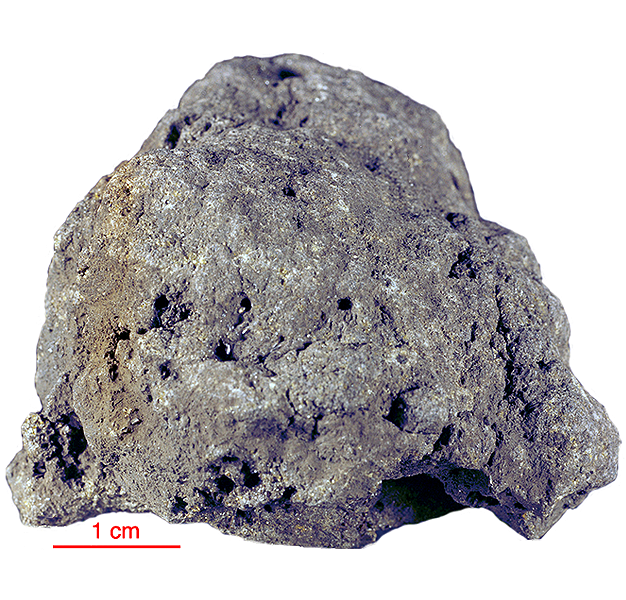This image displays a primarily gray, oval-shaped rock positioned against a white background. The rock, characterized by its multiple pores and rough, grainy texture, exhibits various shades including lighter gray, light blue, and hints of dark brown dirt or rust, notably on its left side. It appears misshapen with chunks missing at the bottom left and bottom right, resembling a sphere that has been elongated. These gaps create a small cave-like formation towards the bottom right. Surrounding the rock is delicate, soft light enhancing its detailed textures, and at the bottom left corner of the image, there is a red horizontal line indicating a 1 cm scale.